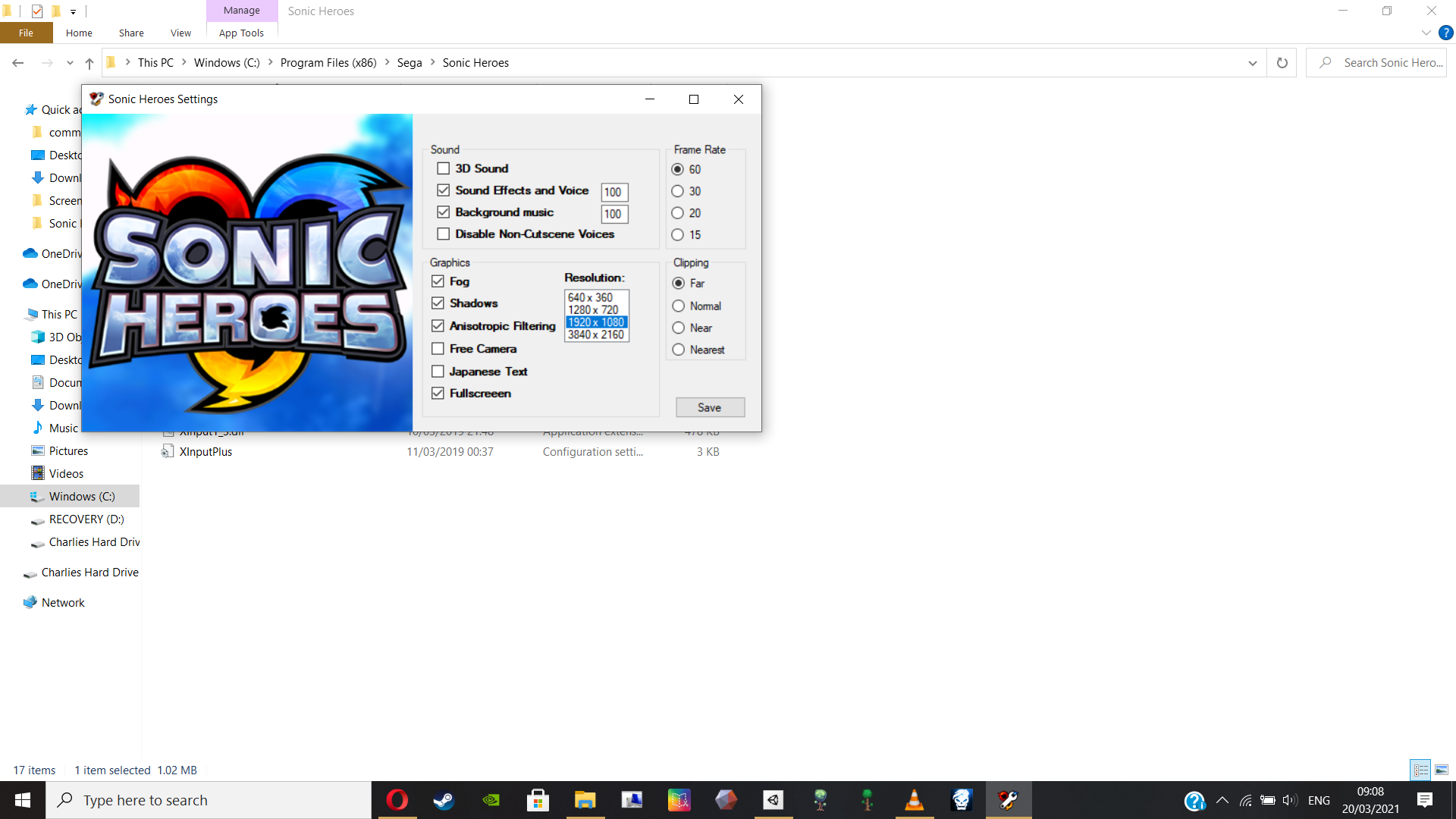The image depicts a File Manager (File Explorer) window on a Windows 10 PC, identifiable from the distinct Windows 10 icons. The taskbar at the bottom of the screen displays several application icons, including Opera Browser, Steam, NVIDIA Control Panel, Microsoft Store, File Explorer, Unity, VLC, and Call of Duty, among others. The main focus within the File Explorer window is a directory path leading to "Sonic Heroes" under "SEGA" in "Program Files (x86)."

Additionally, a game settings menu for Sonic Heroes is open in the foreground, presenting various audio and visual settings. The menu shows:
- Sonic Heroes Settings
- 3D Sound
- Sound Effects and Voice: 100
- Background Music: 100
- Disable Non-Cutting Voices: Not Checked
- Resolution: 1920x1080
- Fog: On
- Shadows: On
- Anisotropic Filtering: On
- Free Camera: Disabled
- Japanese Text: Disabled
- Full Screen: Disabled